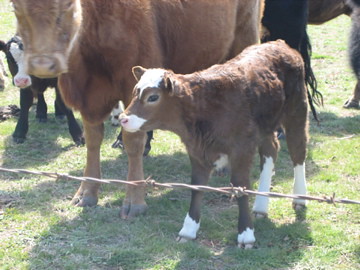A photograph captures a serene outdoor scene on a sunny day, featuring a few cows standing on a green lawn. In the center of the image, a brown baby cow with distinctive white markings—a spot on its forehead, snout, and white feet—stands next to a larger, all-brown cow with grayish feet, though the adult cow's head is cut off at the top of the picture. To the left, another baby cow, mostly black with white on its face and black feet, peeks out from behind the adult cow. The background suggests a hint of more animals, possibly another large brown cow or a horse, visible only by their stomach and hind legs. In the foreground, a brown-grayish barbed wire fence runs diagonally across the picture, with sharp spikes on the wire, adding texture to the rustic setting. The bright sunlight casts clear shadows of the cows on the light green grass, emphasizing the tranquil, sunlit day depicted in the photograph.